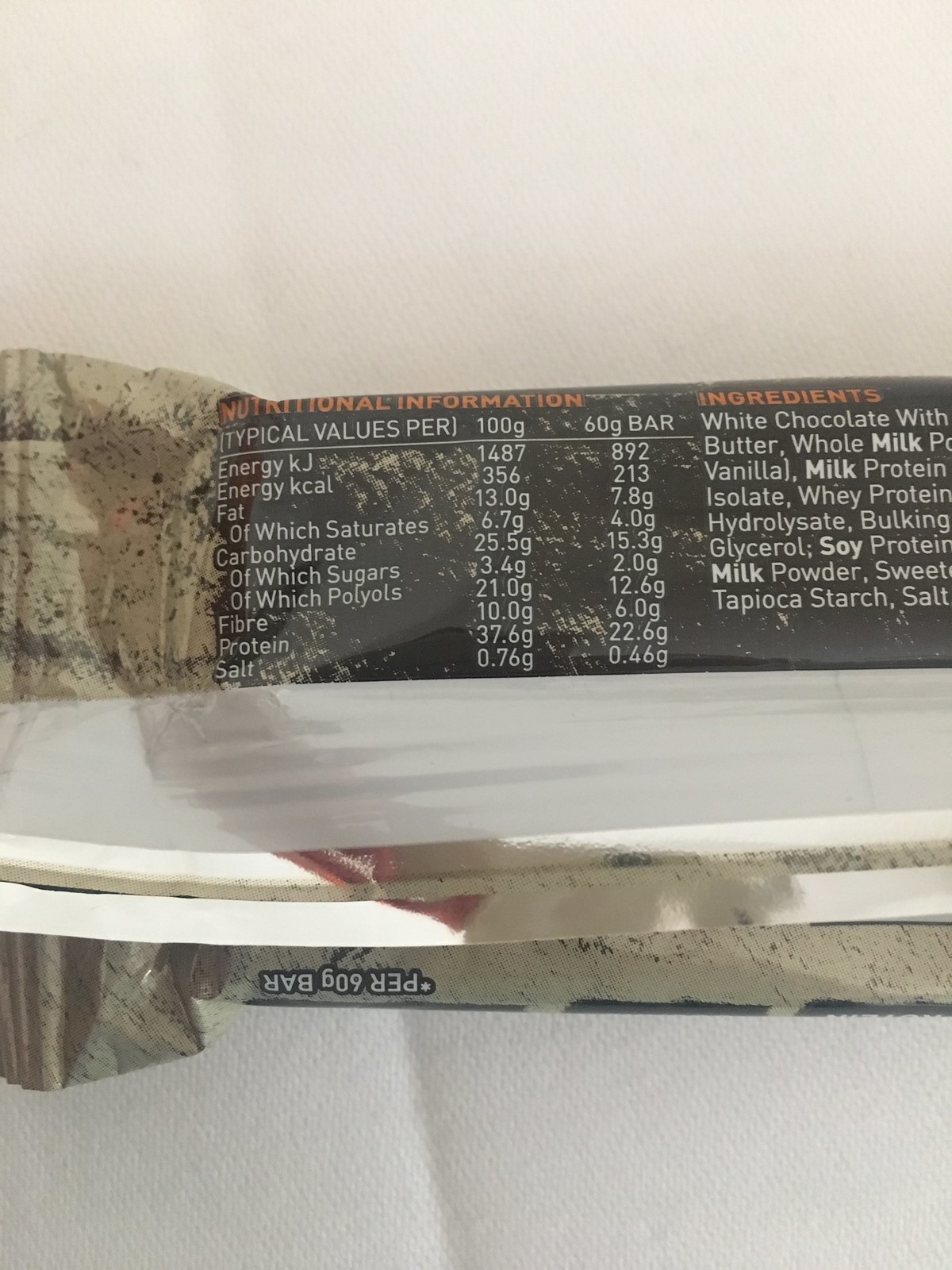The photograph depicts the back side of a partially unwrapped candy bar, positioned horizontally against a textured white background that resembles a paper towel. The packaging of the bar features a metallic silver backdrop with a stone-like texture and black shading, giving it a light brownish-grayish appearance. The focal point of the image is the section displaying the nutritional information and ingredients, which is prominently set against a black background with white text and some silver showing through.

At the top of this section, the words "Nutritional Information" are highlighted in orange. Below this, the nutritional facts are meticulously listed in two columns: one for a 100-gram serving and another for the 60-gram bar. These include detailed values such as energy (1487 kJ/356 Kcal), fat (13.0 grams, of which saturates 6.7 grams), carbohydrates (25.5 grams, of which sugars 3.4 grams, and polyols 21.0 grams), fiber (10.0 grams), protein (37.6 grams), and salt (0.76 grams). 

To the right, the ingredient list begins, marked by "Ingredients" in orange and followed by text in white, with allergens like milk and soy emphasized in bold. The lower part of this informational block transitions to a white bar, beneath which the packaging returns to its original color and texture, indicating the area to peel for opening the bar. However, the lower section of the ingredient list extends off the frame, leaving a portion of it unreadable.